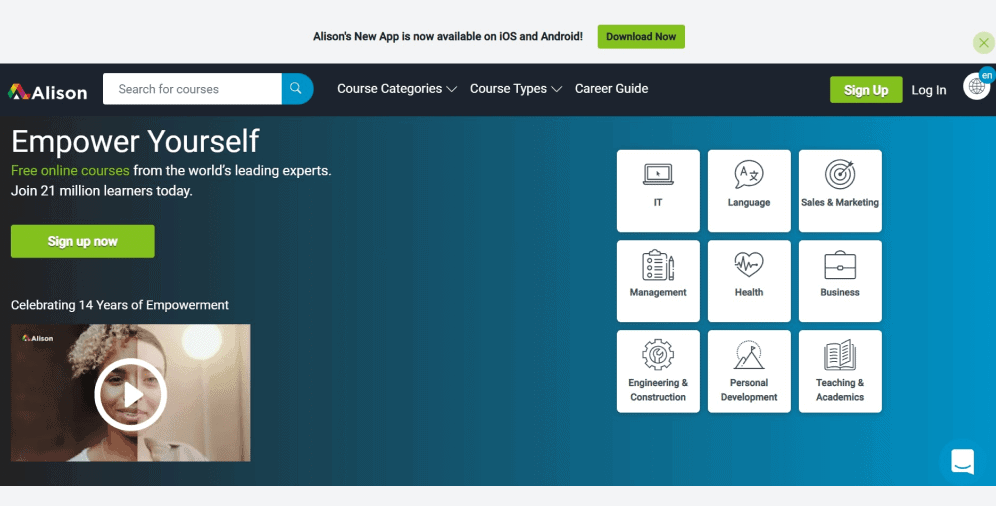The image captures a screenshot of Allison's website, an online course company. At the top of the page, on a black background, there's a prominent menu bar. On the far left is the Allison logo, followed by the company's name in white text. To the right of this is a white search box. Next are the navigation options: "Course Categories," "Course Types," and "Career Guide," each accompanied by a down arrow indicating submenus. On the far right, a green rectangular button with "Sign Up" in white text is visible, next to another white-text link labeled "Log In."

Below the menu bar, a full-width blue background section features a motivational message in various text colors: "Empower Yourself" in white, "Free Online Courses" in green, and "From the World’s Leading Experts. Join 21 Million Learners Today" in white. Centered on this text block is a green rectangular button with "Sign Up Now" in white.

Further down the page, there is a clickable video thumbnail. The thumbnail features an image of two women, seemingly split down the middle. The video icon overlays the center, and above it, white text reads, "Celebrating 14 Years of Empowerment." To the right of the video, there are nine square icons representing different course categories. Each white box with black text and a distinct icon covers a specific field: IT, Language, Sales and Marketing, Management, Health, Business, Engineering and Construction, Personal Development, Teaching, and Academics.